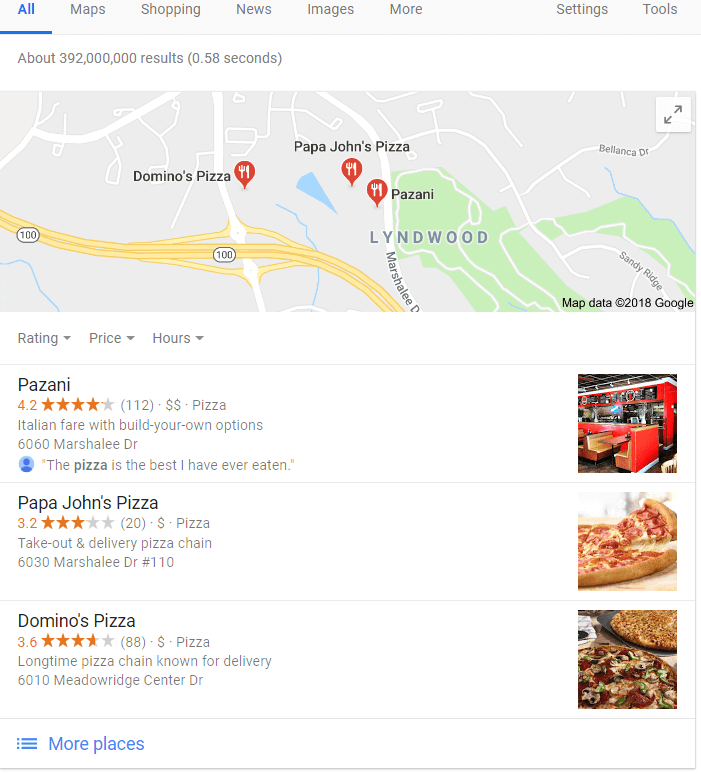**Screenshot Overview of a Google Search for Food**

The screenshot captured from an iPhone reveals a Google search results page, specifically for the term "food." This comprehensive display illustrates a variety of Google functionalities and search results for local eateries.

**Top Section:**
At the topmost portion, the search tabs are visible, including "All," "Maps," "Shopping," "News," "Images," "More," "Settings," and "Tools." The "All" tab is highlighted in blue with an underline, indicating the current view. Below it, there is a note of the search results: "About 392 million results (0.58 seconds)."

**Map Overview:**
The central part of the screenshot features a Google map, showcasing a geographical area of Lyndwood. The map is mostly gray with white roads and a prominent yellow highway (the 100). It indicates three pizza places marked with a red bubble icon containing a white fork and knife:
- **Domino's Pizza**
- **Papa John's Pizza**
- **Paisani**

**Detailed Business Information:**

1. **Paisani:**
   - **Rating:** 4.2 orange stars
   - **Price:** $$ (Moderate)
   - **Description:** Italian fare with build-your-own options
   - **Address:** 6060 Marshali Drive
   - **Review:** The single review is denoted by a blue circle with a silhouette, stating, "The pizza is the best I have ever eaten."
   - **Image:** A red-seated booth with a table and a red pillar, possibly indicating the kitchen area.

2. **Papa John's Pizza:**
   - **Rating:** 3.2 orange stars
   - **Price:** $ (Inexpensive)
   - **Description:** Pizza takeout and delivery chain
   - **Address:** 6030 Marshali Drive, Suite 110
   - **Image:** A slice of cheese pizza being pulled from a whole pie.

3. **Domino's Pizza:**
   - **Rating:** 3.6 orange stars (88 reviews)
   - **Price:** $ (Inexpensive)
   - **Description:** Well-known pizza chain specializing in delivery
   - **Address:** 6010 Meadow Ridge Center Drive
   - **Image:** Two pizzas—one appears to be topped with various veggies like mushrooms, olives, and possibly pepperoni and bell peppers, while the other pizza looks like a traditional cheese pizza.

**Additional Features:**

- **Information Tabs:** Beneath the map are tabs for further filtering by "Rating," "Price," and "Hours."
- **Footer Section:** At the bottom of the map, there is a small text stating, "Map data © 2018 Google." In the upper right corner, there are icons for expanding the view to the left or right. Finally, below the listed restaurants, there's an option labeled "More places" in blue text, providing avenues for further exploration.

This detailed snapshot efficiently conveys various aspects of Google’s local search features and serves as a guide for locating food options in Lyndwood.